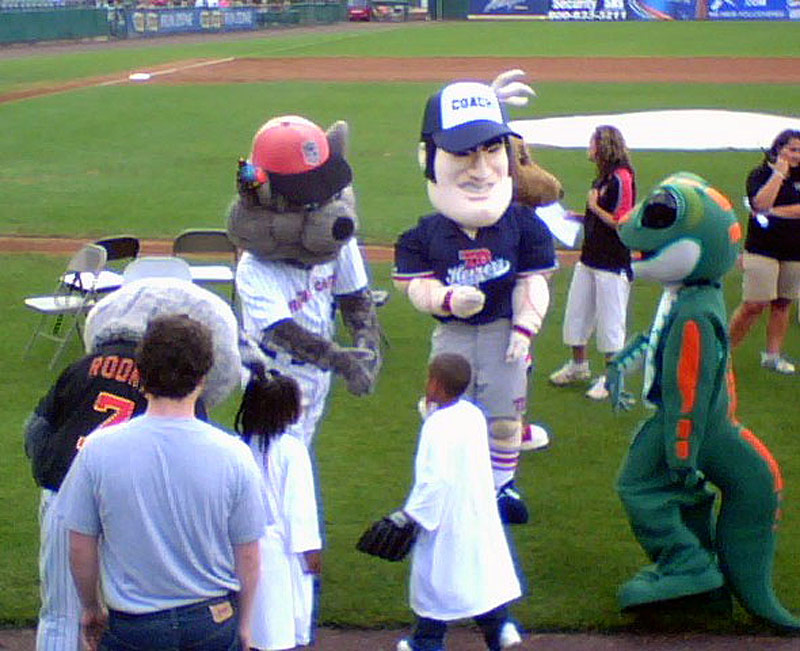The image captures a lively scene on a baseball field where various people and mascots are interacting. The snapshot prominently features a section of the baseball diamond, including third base, and the grassy field. In the foreground, two children wearing oversized white t-shirts are visible, with one child sporting a black baseball glove on his left hand. Surrounding them are several mascots: a lizard-like character with a tail featuring orange markings, a gray coyote or wolf, and a central mascot with a big white face, adorned with a coach's hat in blue and white, bearing the word "Coach", and sporting red and white tube socks, alongside a blue, white, and red jersey.

Among the mascots, there’s also a gray cat wearing an orange hat and a white jersey with red accents. Another mascot bends over nearby, with "ROD" partially visible on its black jersey, along with the red number "7". The scene includes three adults; two are in the background, dressed in shorts and capris, while another man in a light blue shirt and jeans stands to the left. Additionally, there are three old gray chairs positioned to the left side. In the background, beyond the green field, cars in red can be seen with blue and white banners lining the edges of the field, contributing to the lively and colorful ambiance of the event.